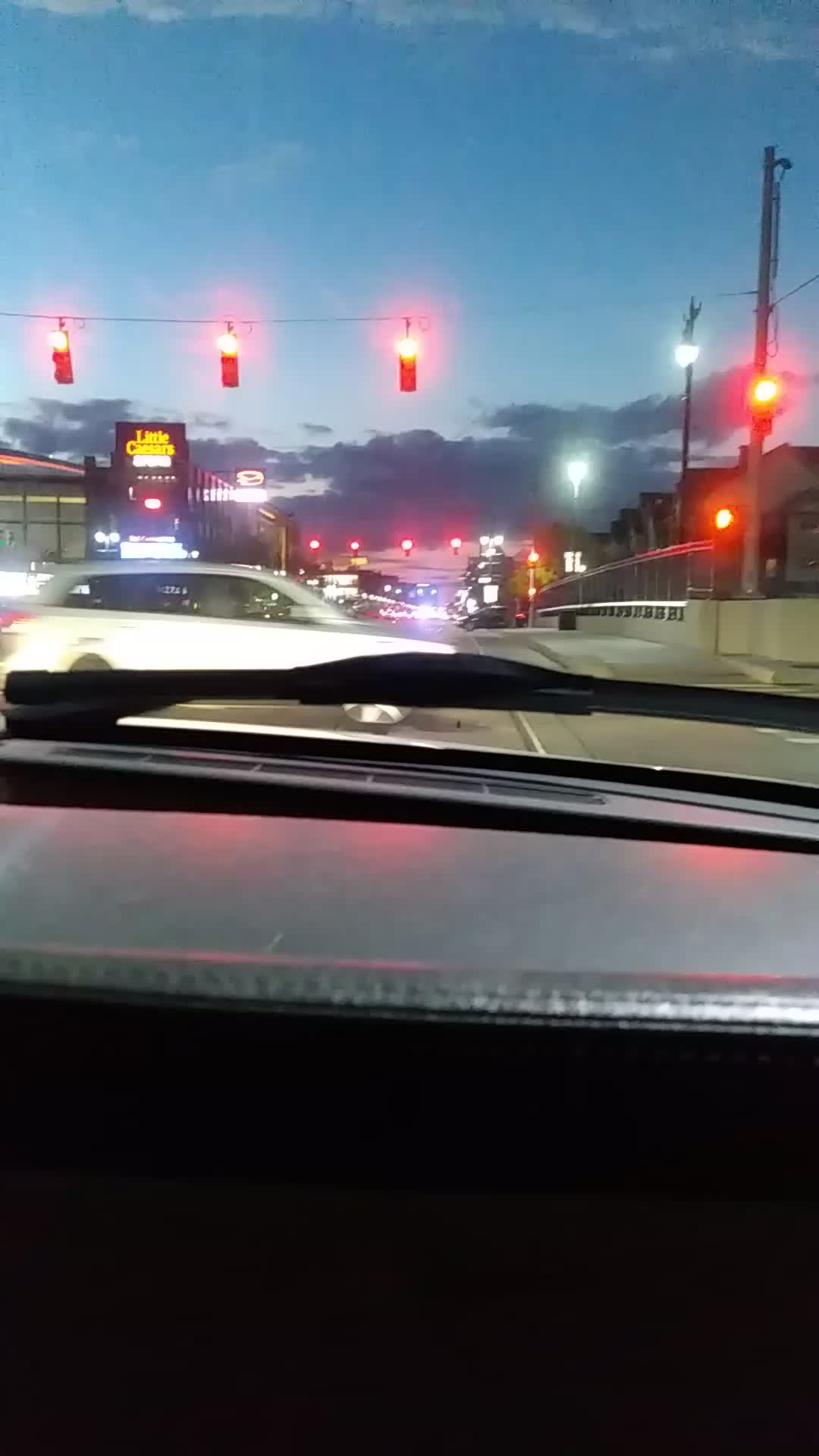The image, taken at dusk from inside a car, captures a scene along a busy street or highway. The backdrop features a dusky blue sky with a few gray clouds. The car’s gray dashboard and black windshield wiper are in the foreground, leading the viewer’s eye towards a red traffic light. A white SUV is driving underneath these lights. The scene is richly detailed with several traffic and street lights dotting the roadway. On the left side, there is a recognizable Little Caesar's Pizza and an Enterprise Car Rental, suggesting a cluster of businesses. Large sidewalks along the street are visible, adding to the urban environment. A bridge with a fence is seen on the right, separating the highway from what appears to be houses or apartments. The various lights in the image have a noticeable bloom effect, enhancing the nighttime atmosphere.